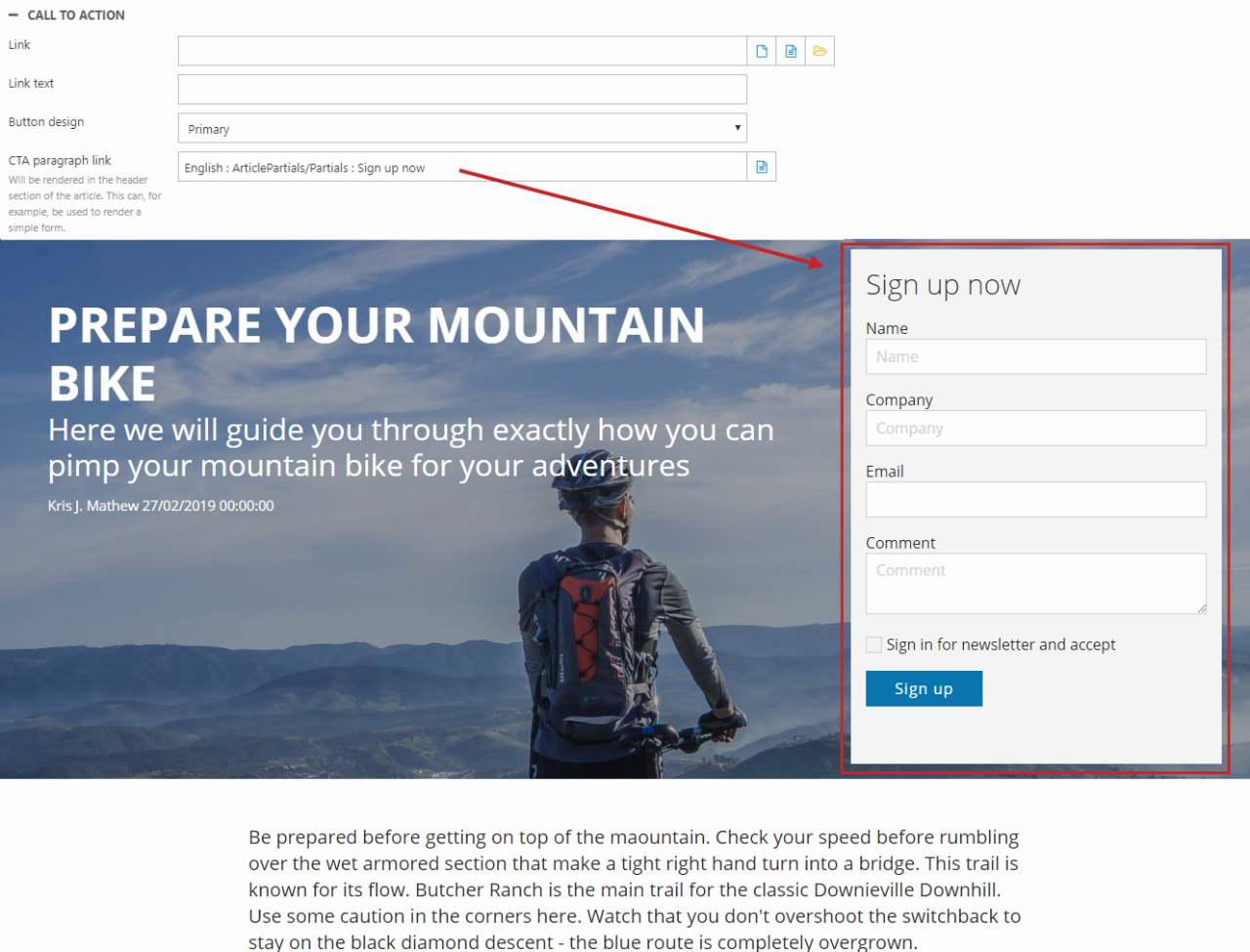The image showcases a user interface for a call to action configuration tool, positioned at the top left corner. The components are detailed as follows:

- At the very top, black text reads "Call to Action." 
- Beneath it, there's a labeled input box for "Link," where users can enter a URL.
- The next item is labeled "Link Text," accompanied by another input box for specifying the text that will appear for the link.
- Below this, you'll find "Button Design" next to an input box pre-filled with the word "Primary." At the far right of this box, there is a drop-down arrow icon in black.
- Under "Button Design," there's another section labeled "CIA Paragraph Link," followed by an input box containing "English: Sign up now." A prominent red arrow extends from this input box, pointing downward towards a white box that also displays "Sign up now."
 
The bottom portion of the UI features a large, visually appealing blue box that serves as a preview area. This background, depicting a blue sky filled with clouds and a picturesque mountain horizon, sets a serene and adventurous mood. The overlaid text reads "Prepare your mountain bike,” followed by “We will guide you through exactly how you can pimp your mountain bike for your adventures,” setting an enthusiastic tone for outdoor enthusiasts.